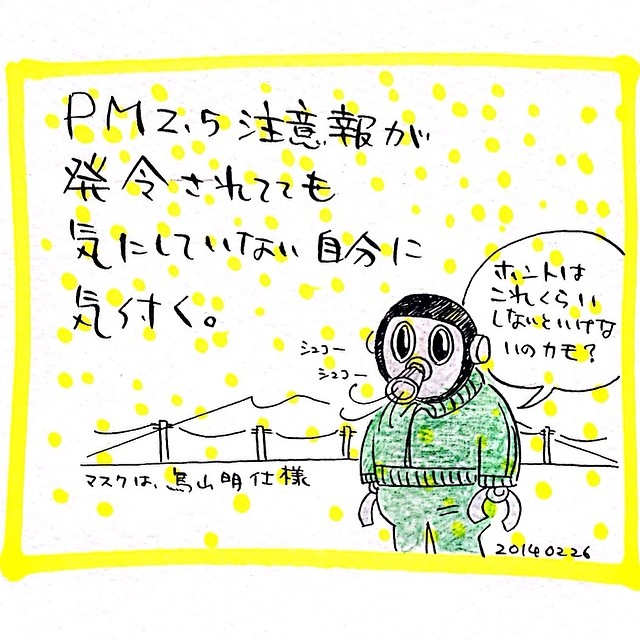This illustration, possibly a comic, features a distinctive character set against a complex background. The main figure, situated slightly to the right, is depicted wearing a green jumpsuit and a gas mask that covers a tight-fitting hood, giving the appearance of a robot or mannequin with steel claw-like hands. The character, drawn in black, white, gray, and green tones, is speaking, indicated by a speech bubble filled with non-English text—likely Japanese—though its exact meaning is unclear. Surrounding the image is a hand-drawn yellow frame, complemented by yellow polka dots scattered over the white background, perhaps symbolizing snow. In the background, details include a bridge or possibly telephone poles and wires stretching across, along with the outline of a mountain. The image also features textual elements in a foreign language on the upper left corner and a numerical date "20160226" at the bottom, within the yellow border, adding to its layered context.